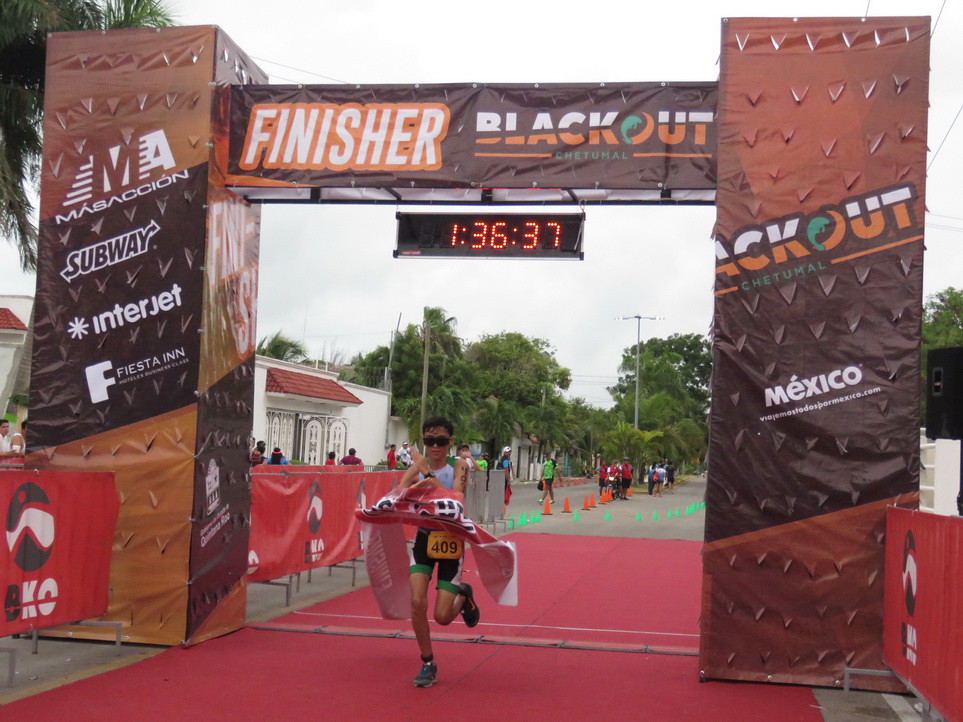In this vibrant outdoor image, a triumphant runner, adorned with the number 409, is captured as he crosses the finish line of a race, holding a torn banner signaling his victory. The scene is set in the middle of the day, featuring a red carpet stretching across an asphalt road, marking the finish line. The finish line structure is notable for its two brown and dark brown columns connected by a bridge-like overhead displaying various advertisements including "Subway," "Interjet," "Fiesta Inn," and prominently "Finisher Blackout" alongside a clock that reads 1:36:37, indicating the runner's time. The runner wears a white shirt and black shorts with a green stripe, centrally positioned in the image, running past the spectators who line the street. In the backdrop, there's a mix of greenery and a white building, with colorful banners adding to the festive atmosphere of the event in Mexico. The colors in the image are vivid, with red, gray, white, black, brown, green, and orange painting a lively scene. Cones are seen set up around the area, highlighting the organized setup of this exhilarating race event.